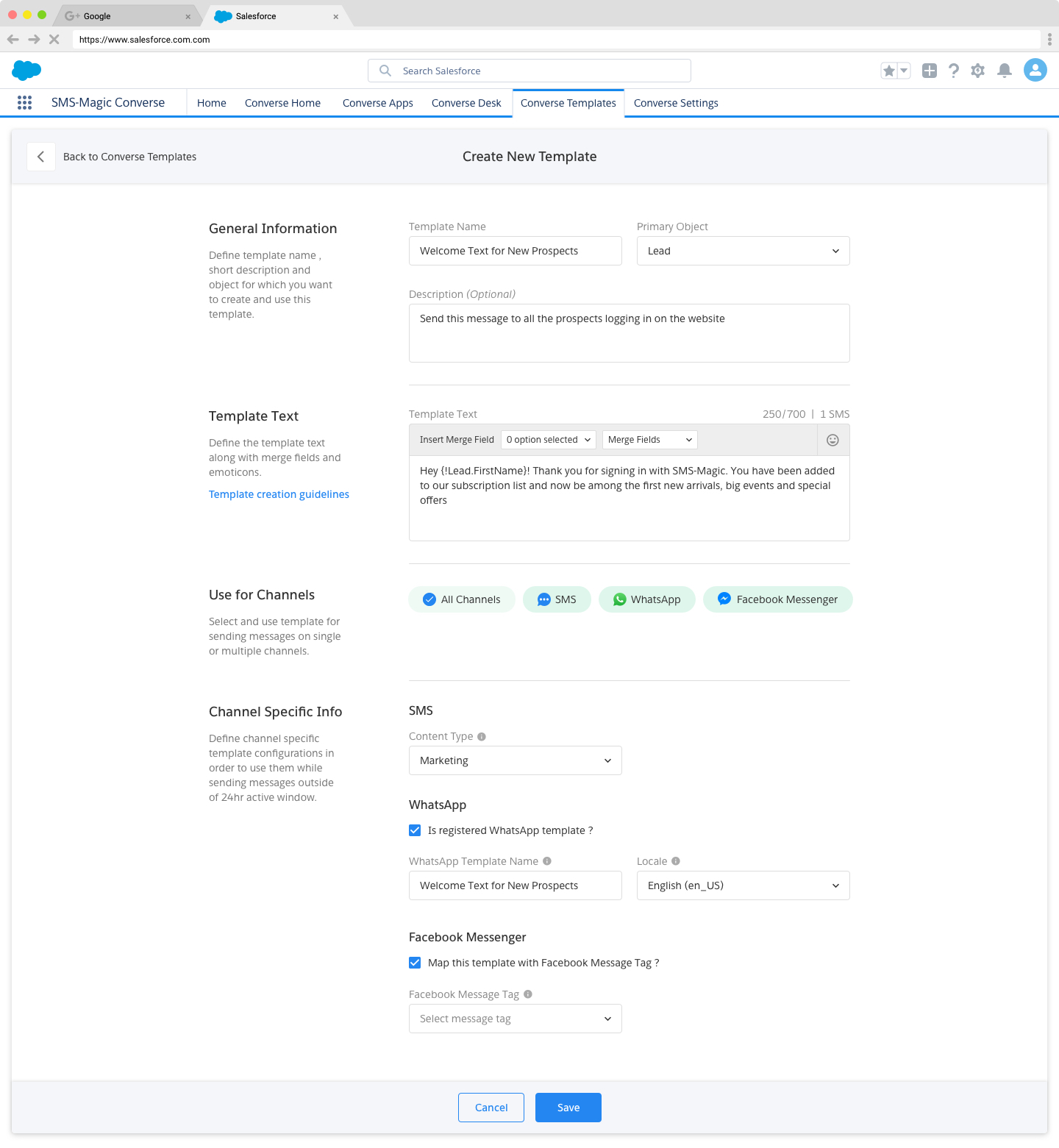This is a detailed screenshot of a web browser interface featuring two open tabs. The first tab is labeled "Google," while the second tab, which is currently active, is labeled "Salesforce." Below the tab bar is the browser's address bar, displaying "https://www.salesforce.com." The address bar also includes standard navigation buttons: back, forward, and an X button for closing the tab.

Directly below the address bar is a gray navigation bar spanning the width of the screen. On the far left of this bar is a blue cloud icon, representing Salesforce. In the center, there is a search field with a gray magnifying glass icon, bearing the text "Search Salesforce" in gray font. On the far right are several functional buttons: one for favoriting items, another for adding content, a question mark for help, a gear icon for settings, a bell for notifications, and an empty profile picture placeholder with a generic white humanoid figure.

Below this navigation bar is another white bar containing several tabs related to specific functionalities within Salesforce: "SMS-Magic Converse Home," "Converse Home," "Converse Apps," and "Converse Desk." This detailed layout showcases the various tools and sections available within the Salesforce interface.